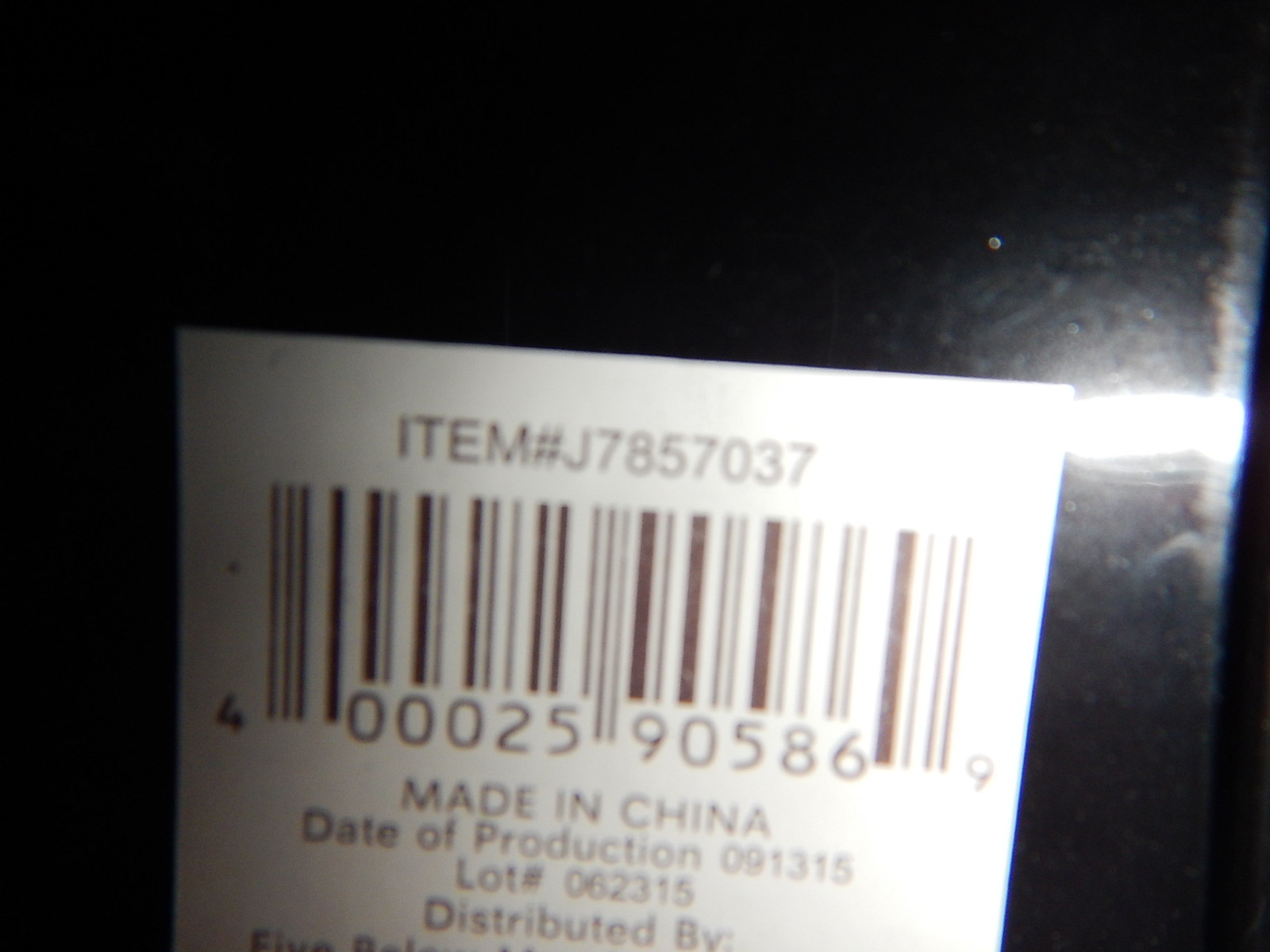In this image, we are viewing the back of an indistinguishable product, rendered entirely in black. The background is equally black, indicating that the picture was likely taken in a very dark room with a flash reflecting off the product. Centered on the product is a prominent white label. This label features an item number and a barcode. Beneath the barcode, text reads: "Made in China, Date of Production: 09-13-15, Lot Number: 062315." The label also begins with the phrase "Distributed by," but the remainder of this information is cut off and unreadable.